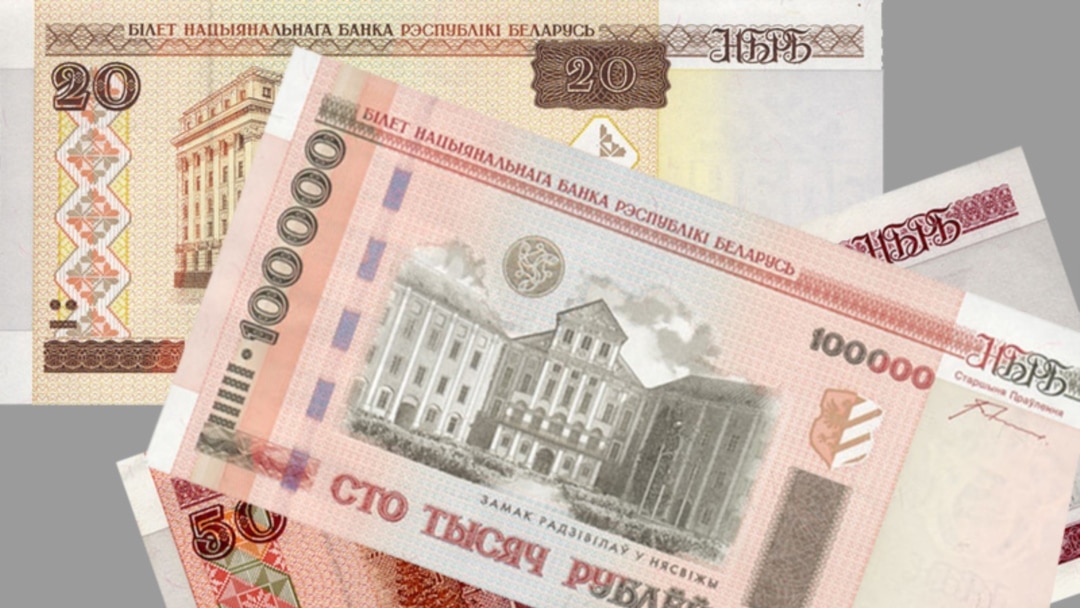This photograph showcases a collection of foreign currency placed against a solid gray background. Prominently displayed are three colorful paper bills, each featuring significant architectural landmarks. The bill in the lower left corner is yellow and valued at 20, with a stately building depicted on it. Above it is a red bill worth 50, partially obscured by the overlapping bills. The most notable bill, on top, is denominated at 100,000 and is distinguished by its intricate design and depiction of an old, stately building. All the bills feature foreign text, possibly indicating their origin from a country with a Cyrillic-based alphabet, such as Russia or a Baltic state.